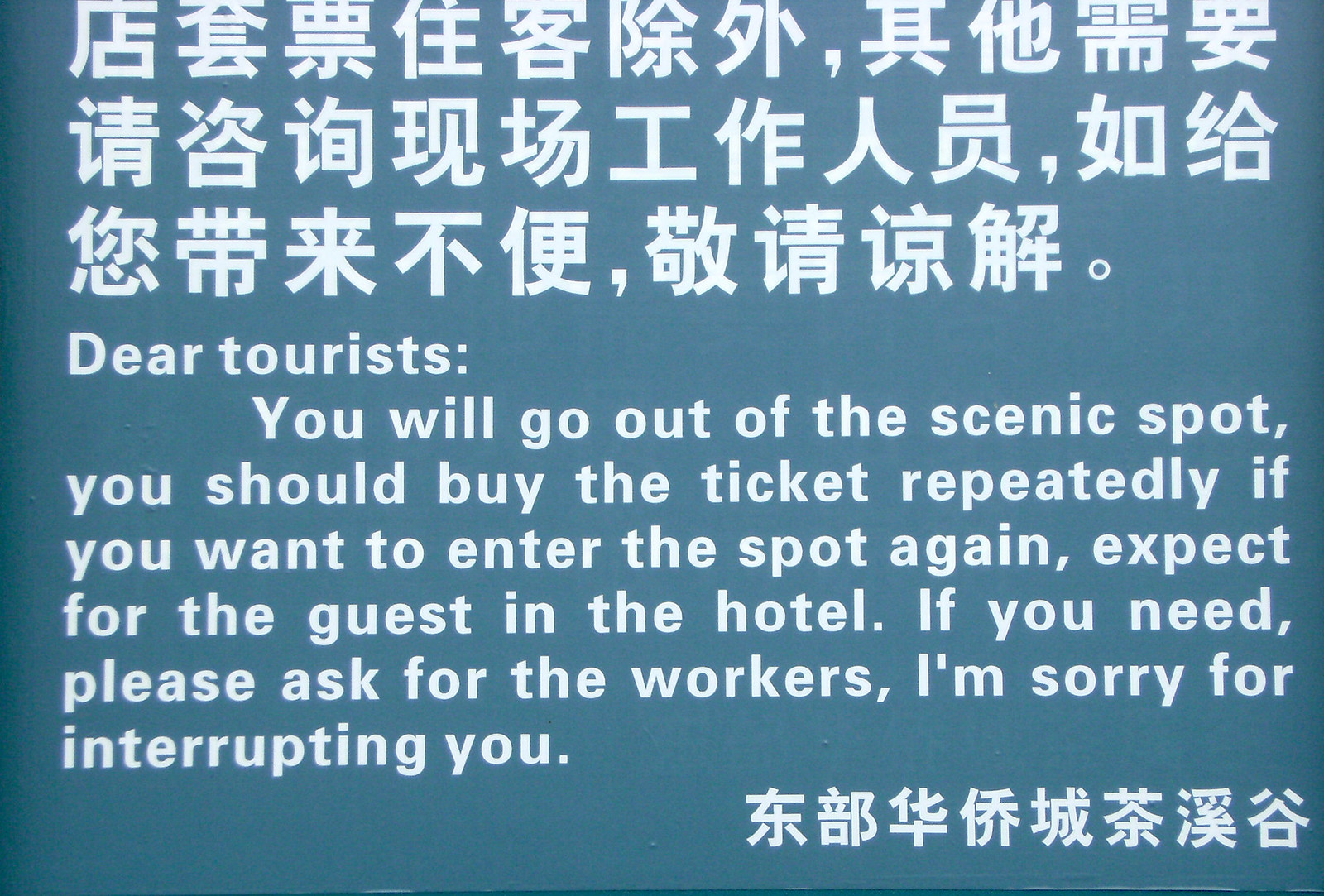The image is a digital screenshot of a sign with a dusty blue or turquoise background. The top half of the sign features white oriental symbols, likely Japanese or Chinese, while the bottom half contains a translation in English. The English text reads: "Dear Tourists, you will go out of the scenic spot. You should buy the ticket repeatedly if you want to enter the spot again, except for the guests in the hotel. If you need, please ask for the workers. I'm sorry for interrupting you." The sign provides clear instructions for tourists about re-entry to the scenic spot, emphasizing the necessity of purchasing a new ticket for re-entry and offering assistance from workers if needed.